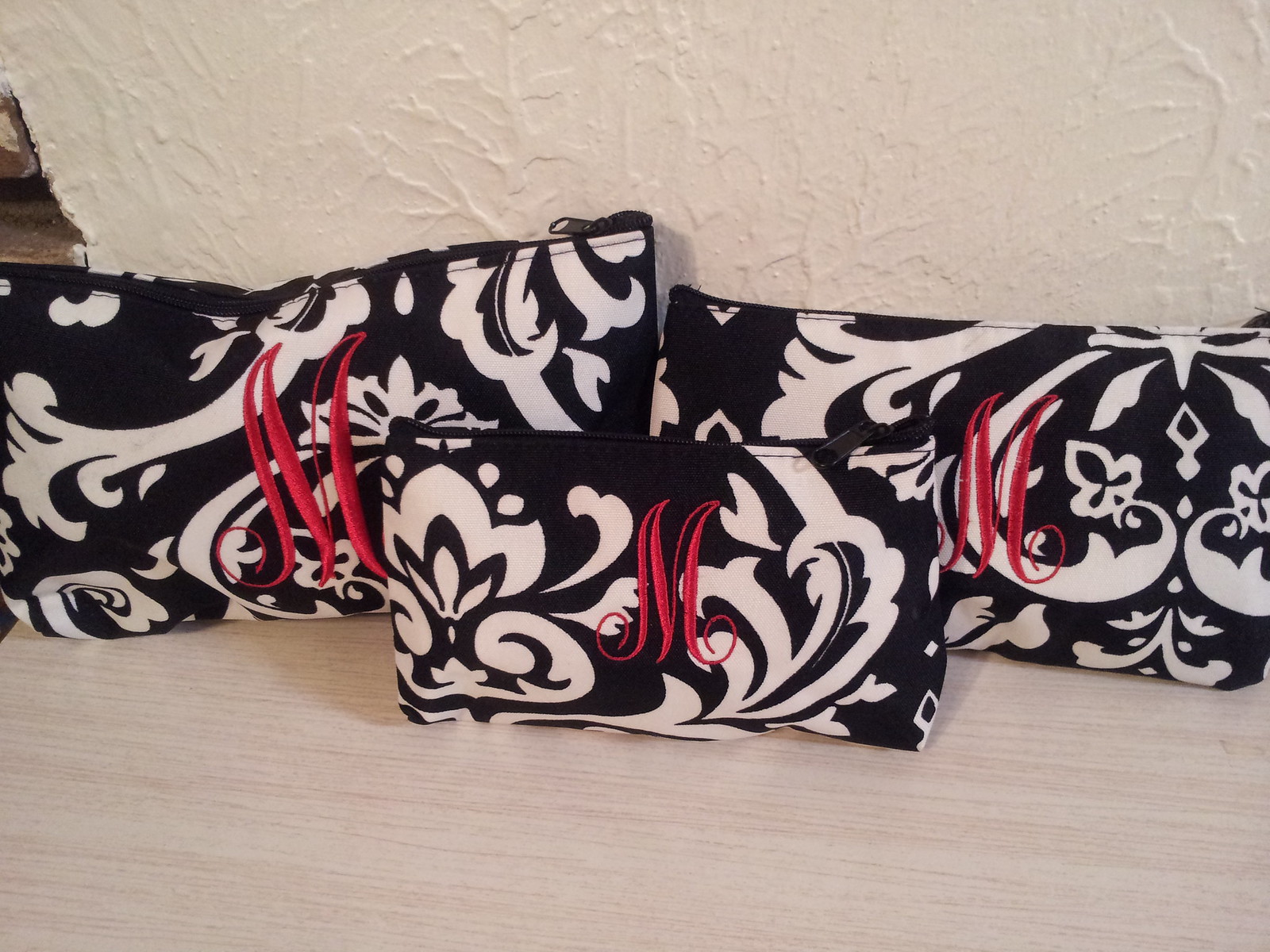The photograph captures three rectangular-shaped items, which are likely either pillows or small pouches, positioned on a beige wooden floor against a textured white wall. Two larger items are at the back, with one slightly smaller than the other, while a smaller item is centered in front of them. Each features a distinct black and white floral design, adorned with various shapes, including arches, heart-like forms, and check marks. Central to each item's design is an embroidered, cursive capital "M" in a hot pink hue. A black zipper is visible at the top of each, with the zipper pull extending to the right. The overall setting includes a mix of elements, notably a floor and wall that provide a neutral backdrop to the visually intricate and colorful designs of the items.